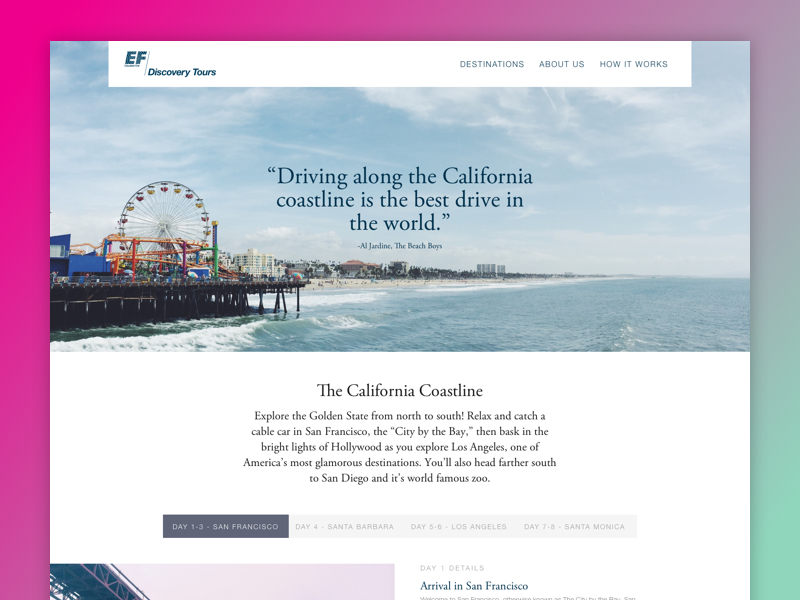The image depicts a borderline website layout, about 20-30% wider than it is tall. The border, occupying approximately 10-20% of the image's width, transitions in color as it progresses clockwise—from a purplish pink in the lower left, shifting to a brighter pink towards the top, transitioning back to purple as it moves right, and finally blending into a sea green along the right edge.

The website header prominently features the initials "EF" in teal, followed by a horizontal bar, with the text "Discovery Tours" also in teal positioned in the lower right of the header. On the right-hand side of the header, menu items labeled "Destinations," "About Us," and "How It Works" are displayed against a white background.

Below the header, a large banner spans the width of the page. The upper 75% of this banner showcases a scenic sky. Below this, on the left side, there's a shoreline featuring a dock, a Ferris wheel, and commercial buildings. The lower right of the banner is dominated by a body of water.

The remaining area beneath the banner has a vast white background, where a centered paragraph of text is situated, providing further details or descriptions.